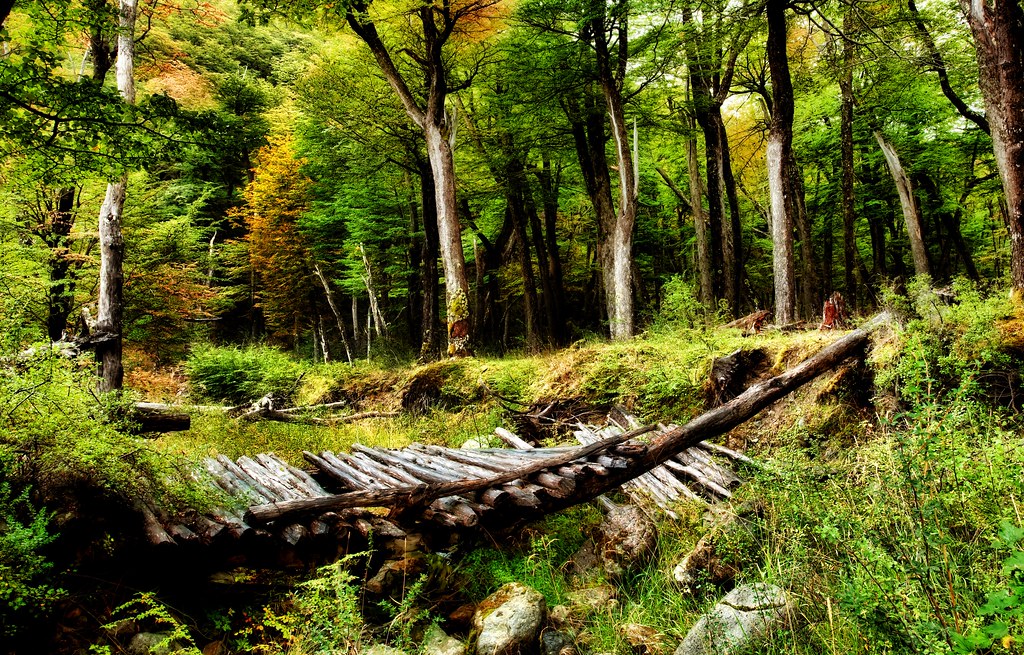In this detailed depiction of an outdoor forest scene—likely a digital creation or a painting—a collapsed wooden bridge takes center stage, positioned slightly below the middle of the image. The bridge, constructed from large tree trunks and smaller branches, appears old and worn, having fallen on its right end into a small ravine or divot devoid of any water. The collapse suggests the bridge might have once served to help people cross this minor ravine. Surrounding the bridge is a lush and vibrant northern forest, rich with greenery and an abundance of small bushes and shrubs, some of which may have moss growing over them. The middle ground features tall trees with brown and white trunks, and pine trees can be seen interspersed throughout. Indications of early autumn are present, with some trees displaying orange and yellow leaves amidst the predominantly green foliage. The scene, rendered in shades of tan, brown, light and dark green, orange, red, and black, captures the serene and slightly melancholic beauty of this secluded, verdant woods.